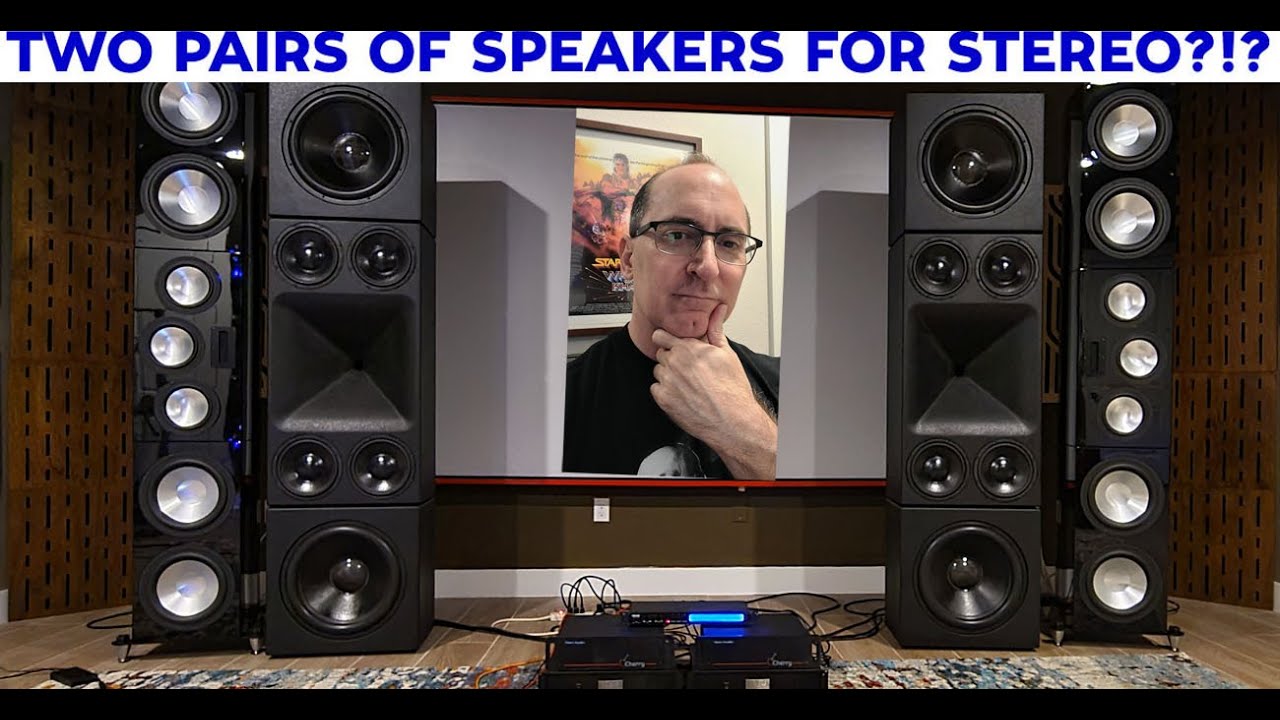The image depicts an elaborate home theater setup featuring a series of sophisticated and large speakers. Dominating the scene, two pairs of substantial black speakers flank the sides of a central projector screen, which displays an image of an older, balding man with glasses, a cleft chin, and a black shirt. He has his thumb resting on his chin and appears to be in his 40s or 50s. The man is shown standing in front of a framed poster — possibly a Star Wars poster from the 2000s — which adds a touch of nostalgia to the setting.

The speakers are notably tall, arranged in stacks with multiple white circular components that resemble subwoofers. There is a total of four massive speakers, some equipped with unique triangular cut-outs. Additional audio equipment, including receivers and amplifiers, sit on the floor beneath the screen, seemingly upon a colorful rug and emitting a blue light, indicative of their active status. The entire setup is framed against a brown wall dotted with black accents, adding a warm and inviting atmosphere to this high-tech entertainment space.